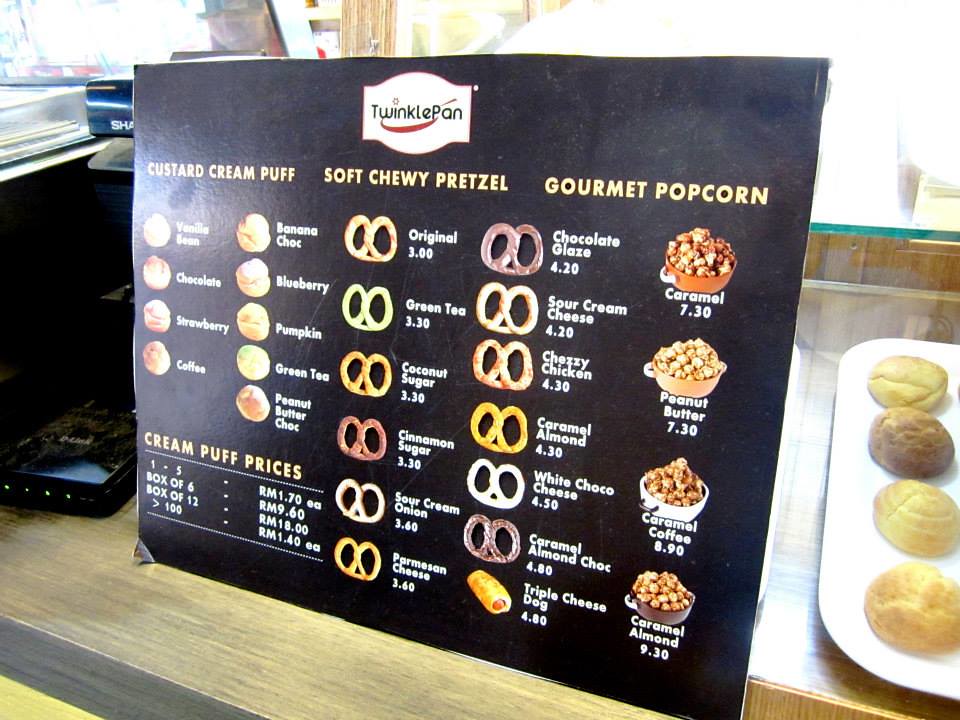The image depicts a well-lit cafe or restaurant displaying a detailed black menu board placed on a brown wooden countertop, positioned behind a glass display case containing bakery items. The menu board, labeled "Twinkle Pan" at the top, is sectioned into three categories: Custard Cream Puff, Soft Chewy Pretzel, and Gourmet Popcorn, each accompanied by corresponding images of the items. The Custard Cream Puff section lists flavors such as Vanilla Bean, Banana Chalk, Chocolate, Blueberry, Strawberry, Pumpkin, Coffee, Green Tea, and Peanut Butter Chalk, with pricing of RM 1.70 each for 1-5 pieces, RM 9.60 for a box of 6, RM 18.00 for a box of 12, and RM 1.40 each for orders of over 100 pieces. The Soft Chewy Pretzel section offers a variety of flavors including Original, Green Tea, Coconut Sugar, Cinnamon Sugar, Sour Cream Onion, Parmesan Cheese, Chocolate Glaze, Sour Cream Cheese, Tasty Chicken, Caramel Almond, White Chocolate Cheese, and Triple Cheese Dog, and their prices range from RM 3.00 to RM 4.80. The Gourmet Popcorn section features options such as Caramel Popcorn, Peanut Butter Popcorn, Caramel Coffee Popcorn, and Caramel Almond Popcorn with prices ranging from RM 7.30 to RM 9.30. Additionally, you can see some other items such as a Wi-Fi router and books on the left side of the counter, enhancing the cozy atmosphere. A staff member is positioned inside the glass display case area where the pastries are meticulously arranged.